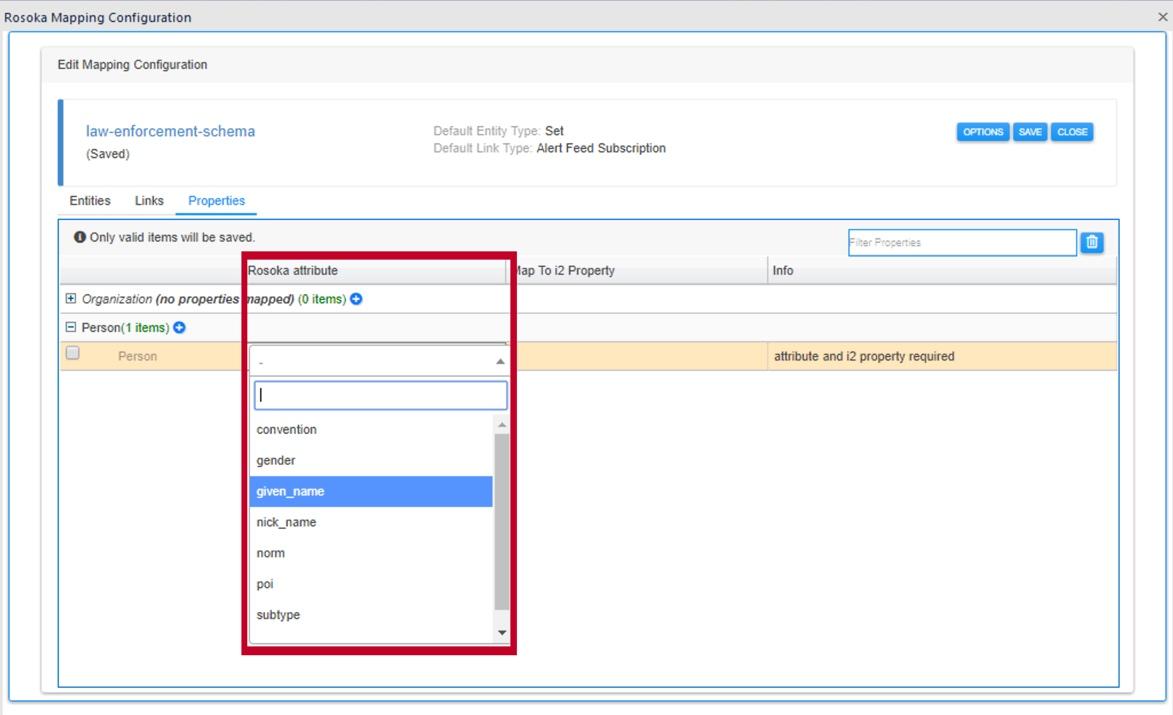This image is a detailed screenshot of a computer screen displaying the "Row SOCA Mapping Configuration" interface. The top left corner of the screen features the title "Row SOCA Mapping Configuration," while the top right corner includes an 'X' button to close the window. Just below the title on the left side, the text "Edit Mapping Configuration" is visible. Underneath that, the screen shows "Law Enforcement Schema" with the word "Saved" in parentheses. The next lines read "Default Entity Type Set" and "Default Link Type Alert Feed Subscription," indicating default settings.

On the right-hand side of the screen, there are three buttons labeled "Options," "Save," and "Close." Beneath these buttons, a notice states, "Only valid items will be saved." Adjacent to this notice is a text box and a trash can icon. The section below lists various categories with corresponding properties: "Organization" with "No properties mapped, 0 items," and "Person" with "1 items." There is a yellow line accompanied by a checkbox next to these items, indicating selectable options.

Superimposed over this section is a vertical red rectangle titled "Row SOCA Attribute." Within this red rectangle, there is a text box for user input, and a dropdown list featuring attribute options such as "Convention," "Gender," "Given Name," "Nickname," "Nom," "Poi," and "Subtype." In this particular instance, "Given Name" is highlighted in blue, although part of the content appears to be incorrectly included within the rectangle.